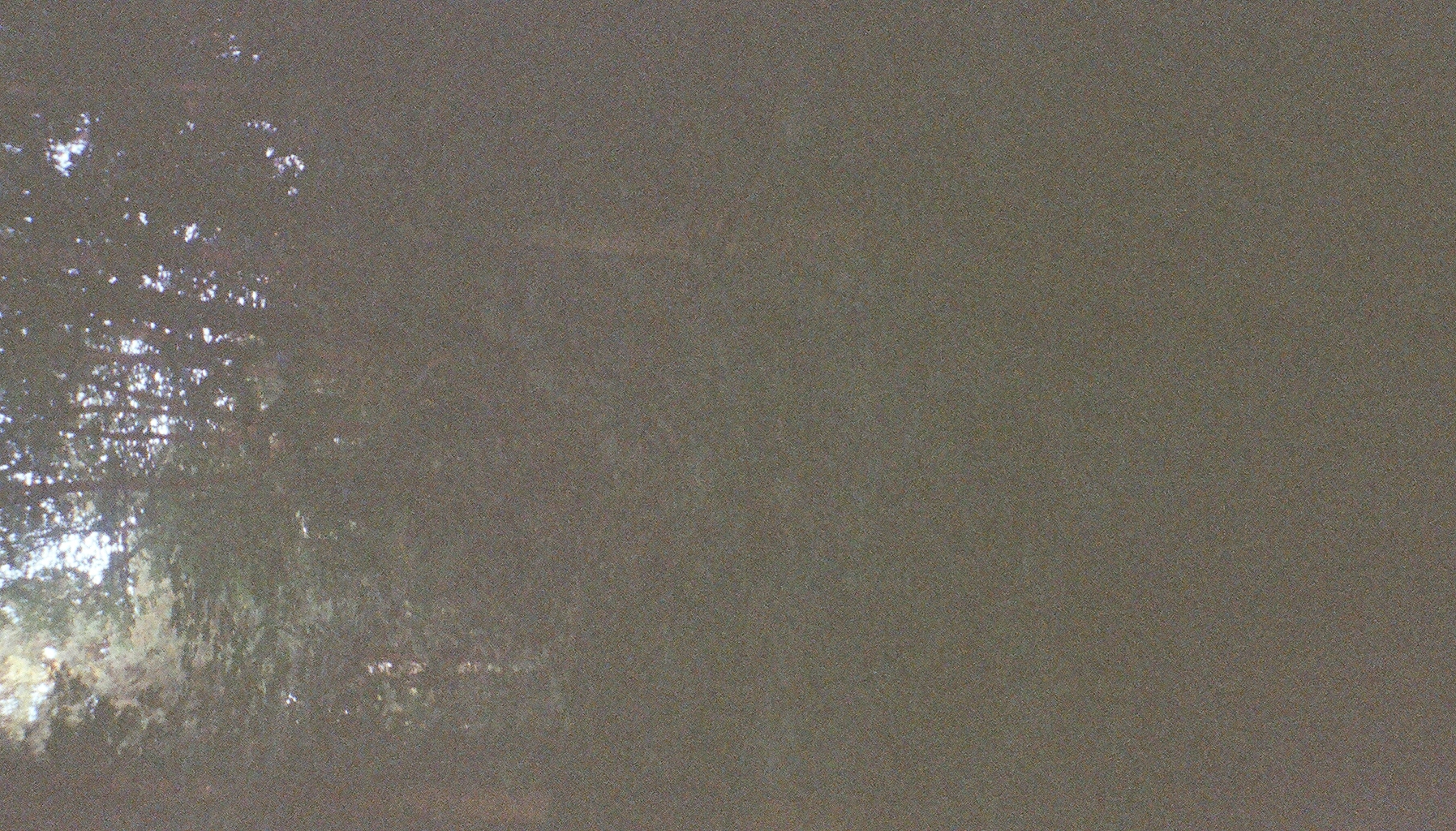The photograph appears to be taken in an outdoor setting, possibly a backyard or a forest, with the orientation of the image being slightly tilted. The overall quality is low, resulting in a hazy, pixelated, and washed-out appearance. The right-hand side of the photo is dominated by dark, almost black sections with notable static-like artifacting and minimal discernible detail. As your eyes move toward the middle, the image begins to reveal more features, including some indistinct tree trunks and branches. Most of the detailed elements are concentrated on the left-hand side, where the sunlight filters through, illuminating the scene. This area displays a vibrant mix of green foliage, suggesting a heavily leafed tree, possibly a willow or weeping willow, with branches interspersed through the bright blue sky. Elements of underbrush and smaller bushes are also visible, enhancing the lush and verdant feel of the environment. The overall setting and the clear blue sky indicate that the photo was likely taken on a bright sunny day during spring, summer, or early fall.